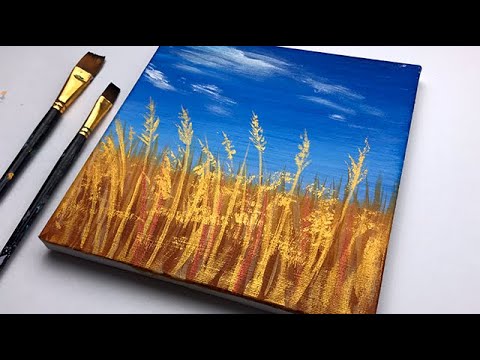This image showcases a detailed painting of a serene wheat field set against a vivid, blue sky with light clouds forming in the top left corner. The painting, resting on a white background, is framed by wide black bars at the top and bottom, giving it a cinematic feel. In the foreground, golden amber and various shades of brown depict the wheat, with distinct yet subtle strands and heads catching the sunlight. To the left of the square canvas, two clean paintbrushes lay side by side, one slightly smaller than the other. Both brushes have gold ferrules and black handles, adding a touch of elegance to the scene.